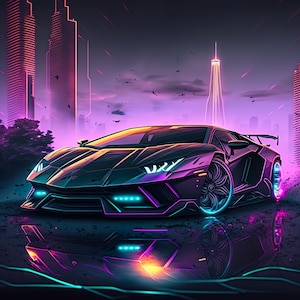This highly detailed digital drawing showcases a sleek, purple two-door sports car, possibly a Lamborghini, with a low profile and a distinctive tapered front hood that gives it a sharp, shark-like appearance. The car features vibrant LED lights underneath and neon turquoise headlights, paired with black and green tires that look almost animated. The back wheel is shown spinning dirt, indicating rapid movement, while the car sits on a shiny black surface that reflects its streamlined form.

In the background, a triangular skyscraper with an antenna at its peak is glowing with neon white light, reminiscent of well-known tall buildings like the one in Seattle, Washington. To the top left of the image, two cylindrical skyscrapers can be seen, alongside black spots in the sky that may be birds. Additionally, a bush with green and black hues is located to the left of the car's hood. The night sky behind the scene is a deep purple with scattered clouds, adding to the dynamic and futuristic atmosphere of the graphic.